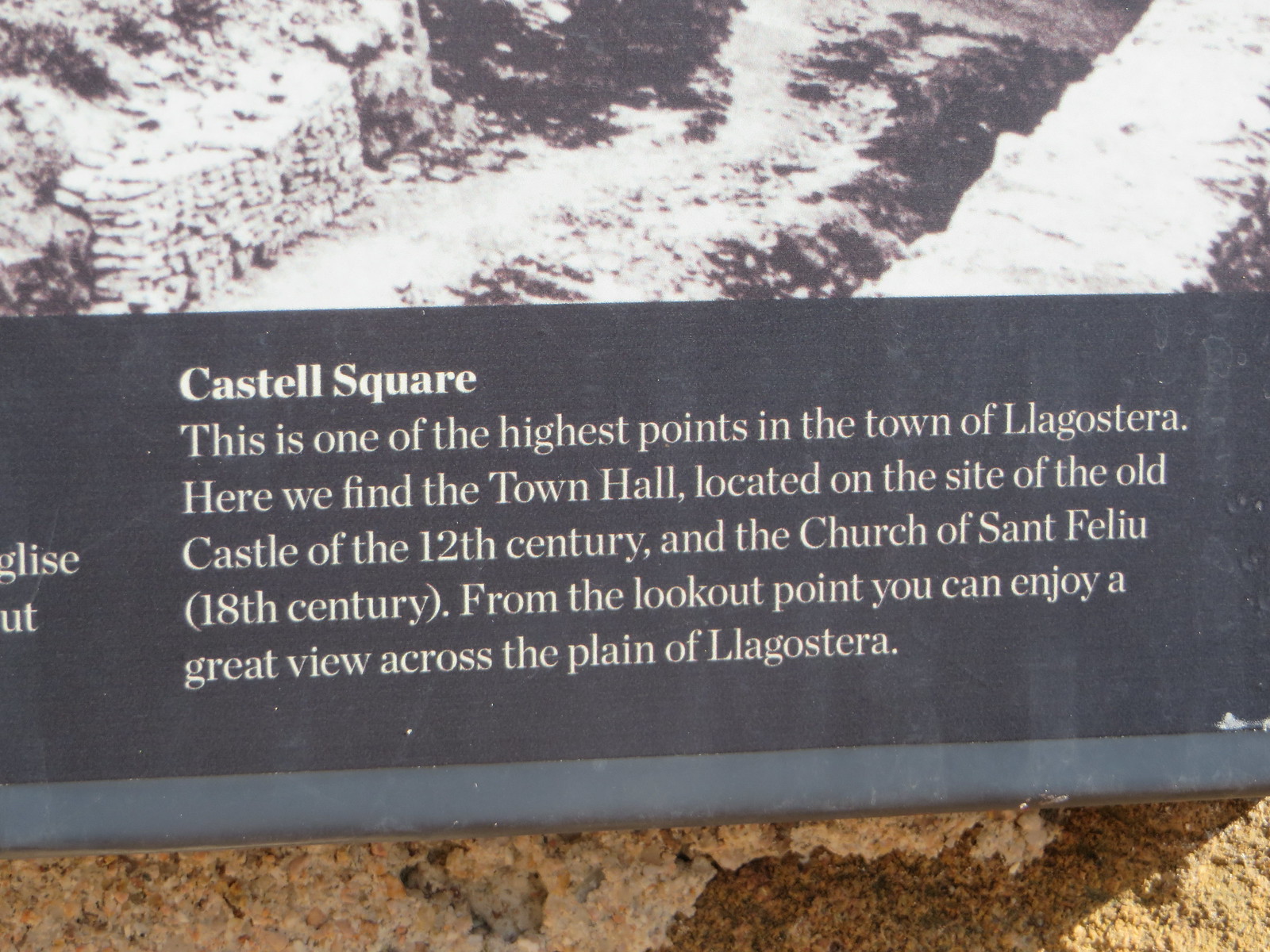The image depicts the bottom portion of an informational sign likely located outside, possibly at a museum or historical site. The sign features a black and white photograph at the top, which appears to depict archaeological remains of a foundation or stone wall. The visible section of the sign's textual content, written in white on a black background, reads:

"Castell (or Castel) Square. This is one of the highest points in the town of Lagostera. Here we find the town hall, located on the site of the old castle of the 12th century, and the Church of Saint Feliu (18th century). From the lookout point, you can enjoy a great view across the plain of Lagostera."

The sign is situated on a rock or stone wall, with the rock's texture and coloration visible around the edges, displaying beige and brown hues. The text and photograph are framed, with additional cut-off words seen on the right side of the sign, though they are not fully legible.